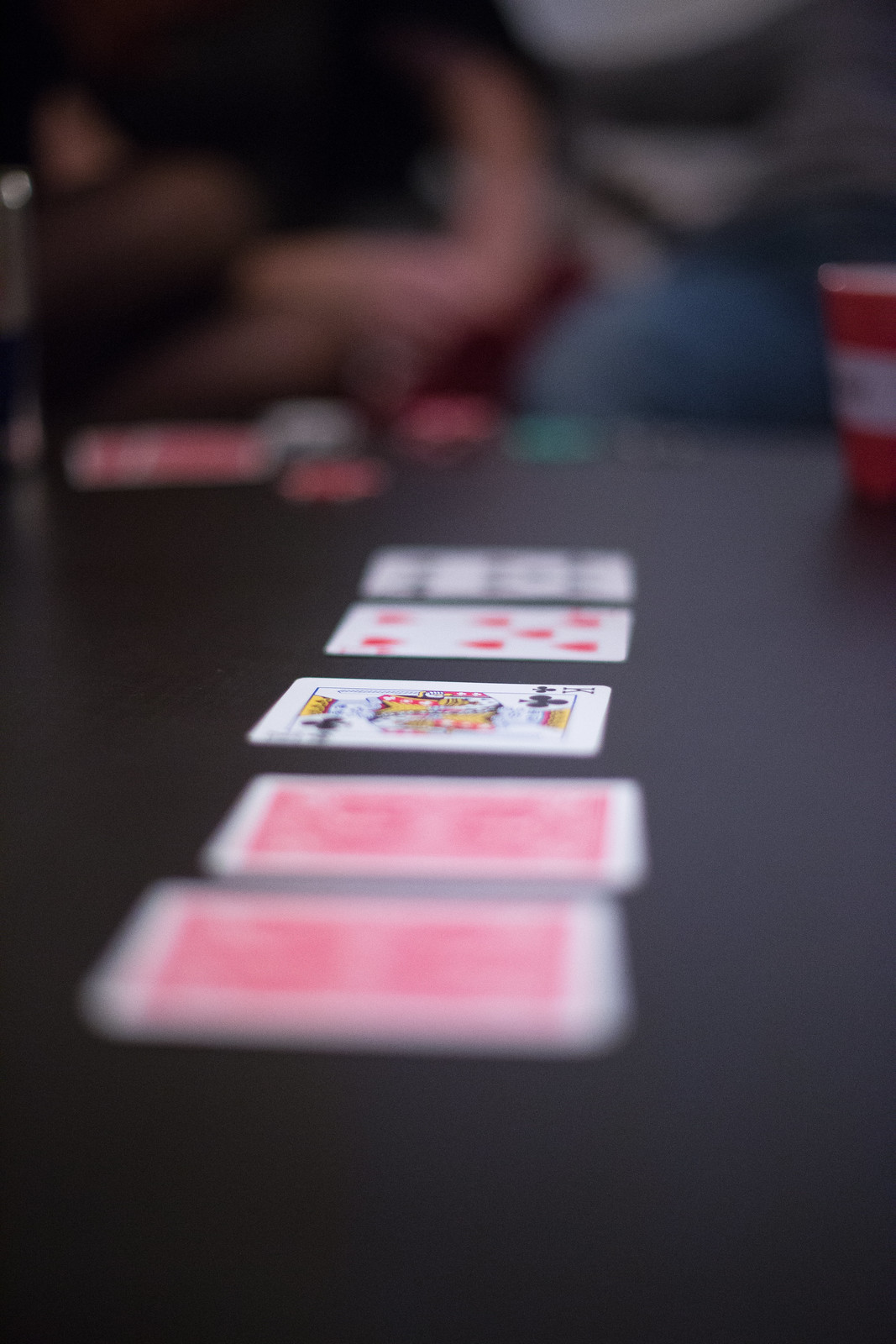In this engaging image, players are engaged in a game of Texas Hold'em poker at a sleek, black table. The table is impeccably clean, devoid of any scratches. In the foreground, two cards are visible but out of focus; the card backs exhibit a predominantly pink color with a white outline. The center of the table features a clearly visible King of Spades and a Seven of Hearts, while the last card on the far end is also out of focus but shows black colors. 

To the right, a red cup with a white label stands prominently. In the background, blurred figures suggest the presence of other players, though their details are indiscernible. On the left side, a slightly upraised arm and elbow can be spotted. Poker chips in stacks of pink and green, alongside a deck of cards, add to the authentic poker night ambiance, though they too are blurred. Additionally, a white item extends slightly from the left stack of cards towards the right, capturing a subtle motion in the scene.